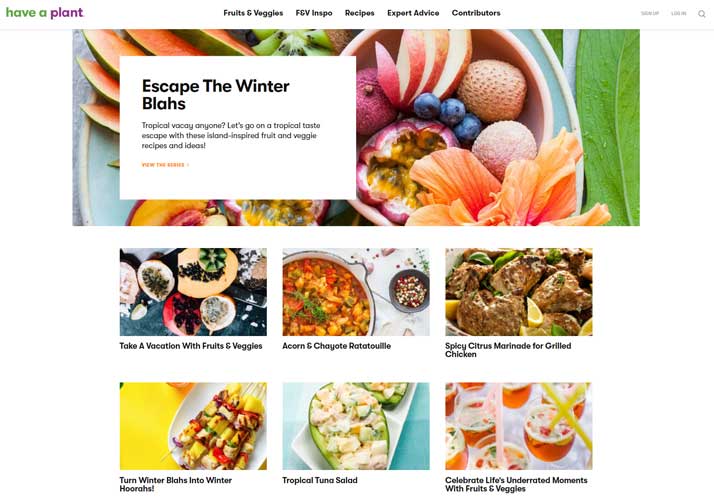The image depicts a vibrant and colorful website titled "Have a Plant," prominently featuring an array of fresh fruits and vegetables. At the top, the website header includes a banner with the text "Fruits and Veggies," and several tabs labeled "FGV and INSPE," "Recipes," "Expert Advice," and "Contributors." The central section showcases a plate brimming with an assortment of colorful fruits, such as blueberries, cantaloupe, watermelon, and greens. An eye-catching orange flower with a green leaf to its right adds a touch of floral elegance.

A playful caption reads, "Escape the Winter Blaze, Tropical Vacay Anyone? Let's Go on a Tropical Taste Journey with These Isle-Inspired Fruit and Veggie Recipes and Ideas." At the bottom, a semi-transparent red-orange pop-up box appears with text that is partially unreadable.

Beneath the main section, there are six smaller, vividly colored boxes featuring different recipes and ideas:

1. "Take a Vacation with Fruits and Veggies" – Promoting a variety of fruity treats.
2. "Acorn and Chayote Ratatouille" – Highlighting a savory vegetable dish.
3. "Spicy Citrus Marinade for Grilled Chicken" – Offering a tangy marinade recipe.
4. "Turn Winter Blaze into Winter Hurrahs" – Showcasing succulent shish kebabs.
5. "Tropical Tuna Salad" – Presented in a halved avocado.
6. "Celebrate Life's Underappreciated Moments with Fresh Fruits and Veggies" – Encouraging the use of fresh produce to enhance everyday experiences.

The overall aesthetic is lively and inviting, with a strong emphasis on fresh, healthful eating inspired by tropical flavors.